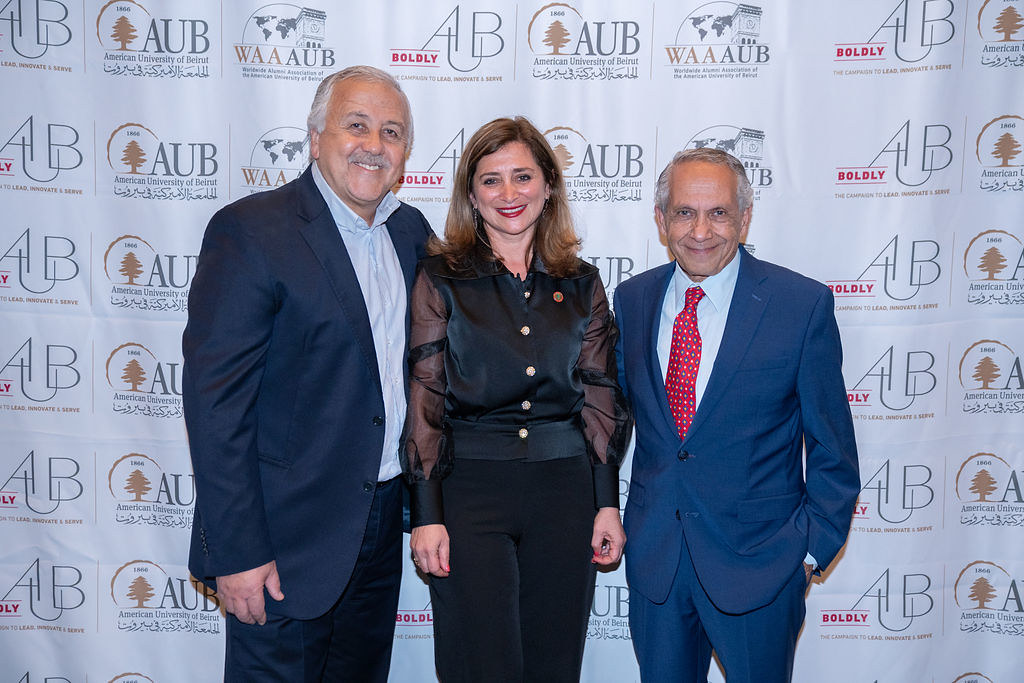In the photograph, three people stand side by side, smiling directly at the camera, in front of an indoor backdrop adorned with a repeating pattern. The backdrop features bold text reading "AUB" and "WAAUB" along with logos from the American University of Beirut, including a blue silhouette of a tree and elements suggesting a globe.

The individuals are centered in the image, with a well-dressed gentleman on the left wearing a dark blue suit paired with a light blue button-down shirt. He sports a mustache and appears to be in his 70s. The woman in the middle, smiling warmly, has dirty blonde hair and is dressed in a black button-down shirt and black pants. She looks to be in her late 30s to early 40s. To her right is an older gentleman, also roughly in his 70s, donning a light blue suit, a light blue button-down shirt, and a red patterned tie.